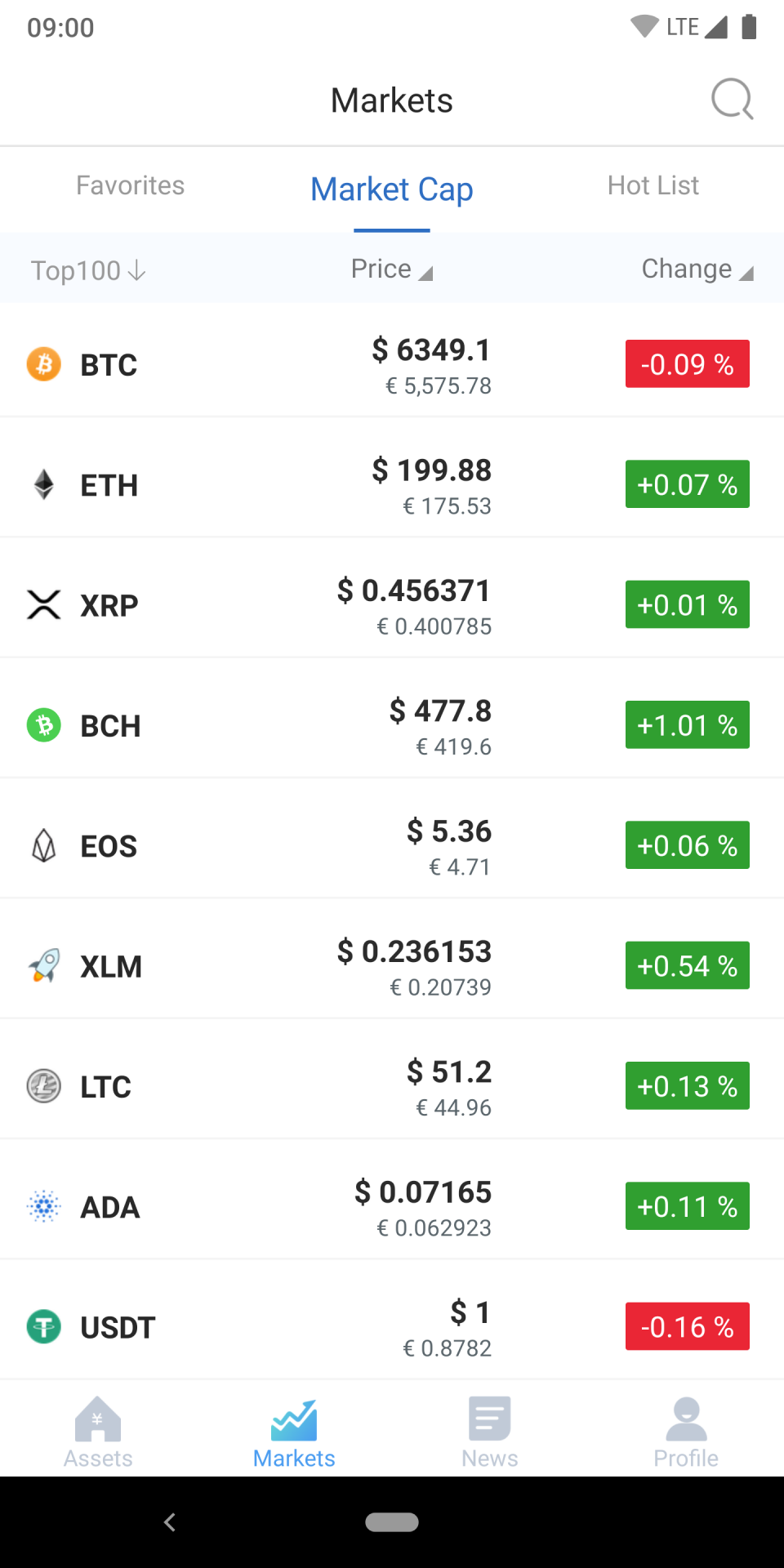This is a detailed descriptive caption for the provided image:

---

The image is a screenshot from a mobile app, featuring a clean white background. At the top-left corner of the screen, the time is displayed as "9:00." On the top-right corner, indicators show LTE connectivity, a Wi-Fi icon, a full mobile signal icon, and a fully charged battery icon.

Below these indicators, the screen displays the word "Markets" in black font. Underneath this, there is a small gray dividing line. Following this, a navigation bar presents several options: "Favorites," "Market Cap," and "Hot List." The "Market Cap" option is currently selected, indicated by blue text and a small blue line beneath it.

Further down, there is a header row within a light gray rectangle that sets the labels for the columns below. These labels are "Top 100," "Price," and "Change."

The "Top 100" column starts with the cryptocurrency abbreviations in the following order: BTC, ETH, XRP, BCH, EOS, XLM, LTC, ADA, and USDT. Correspondingly, the "Price" column lists the current prices in USD for these cryptocurrencies as follows: $6349.1, $199.88, $0.456371, $477.8, $5.36, and $0.236153. 

---

This caption provides a clear, well-structured description of the image, ensuring all details are articulated comprehensively.